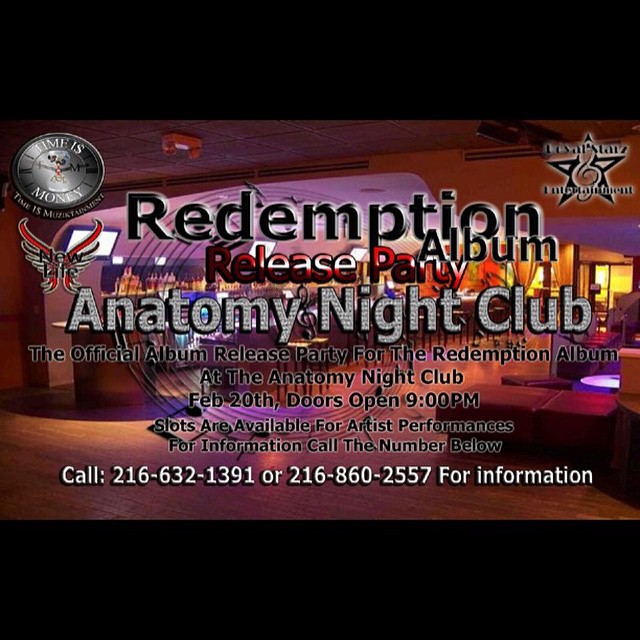The image features a detailed graphic design advertising the "Redemption Album Release Party" at Anatomy Nightclub. Dominated by shades of dark red, pinkish, lighter red, and purple, the sign lays out essential event information in a mix of black, gray, and white lettering. The primary text reads: “Redemption Album Release Party” in black, “Release Party” in red, “Anatomy Nightclub” in a bejeweled silver color, and includes further details—such as "The Official Album Release Party for the Redemption Album at the Anatomy Nightclub," occurring on February 20th with doors opening at 9 PM. Additionally, it announces that slots are available for artist performances and provides contact numbers for more information: 216-632-1391 and 216-860-2557.

The background subtly features the nightclub setting, showcasing a central bar area with lounge chairs and seating, mainly visible at the bottom right of the image. Above the bar, an off-white ceiling transitions to a lowered ceiling towards the back, and three televisions are partially obscured by the overlaying text. The image also includes two logos: one circular silver clock with the inscription "Time is Money" and another featuring a star with a music symbol inside, surrounded by small, unreadable text. Black rectangular borders frame the top and bottom of the image.